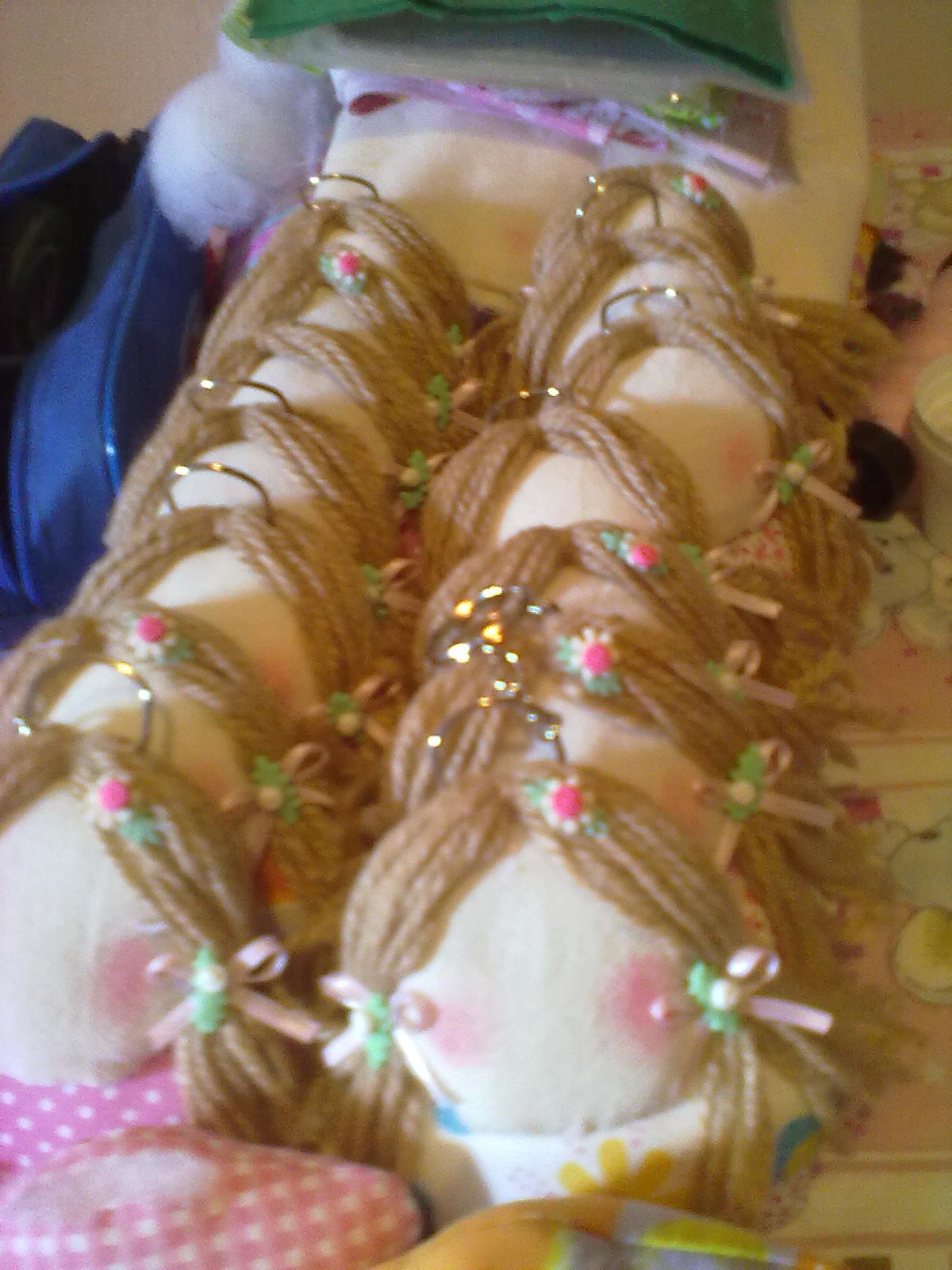In this highly detailed close-up image, we see a collection of unfinished ragdolls arranged in two rows, each at various stages of completion, leaning against each other and a large wool blanket with a multicolored pastel bedspread. The dolls, about a couple of inches high, feature brown or blonde string-like hair adorned with colorful bows, typically yellow and green. Their faces, still to be finalized, appear mostly blank or blushed with the promise of further detailing. Each ragdoll is dressed in a unique outfit, including pink and white dotted dresses and shirts with yellow and blue insignias. Surrounding the dolls, there are blue and green fabric bags, alongside a blue suitcase placed on the floor. In the background to the right, a light brown and yellow drawing or painting can be seen on the wall, adding to the whimsical atmosphere of the scene.